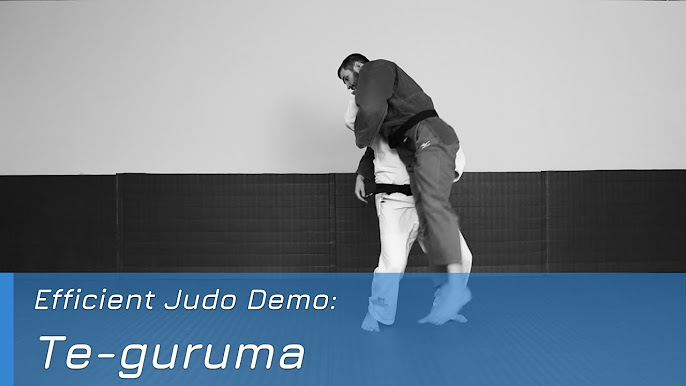In a dojo setting, an image captures two men engaging in a dynamic Judo demonstration. The scene features a room with a white wall and a black padded lower section, indicative of a traditional martial arts training environment. One man, dressed in a white Judo uniform with a black belt, is lifting another man over his shoulder. The second man, clad in a darker gray Judo outfit with a black belt, has short black hair and a short beard, and appears to be mid-air, demonstrating a self-defense technique. Both men are involved in a move known as "Te Guruma," a classic Judo throw. Across the bottom portion of the image, a blue rectangular banner displays the text "Efficient Judo Demo Te Guruma" in white, emphasizing the instructional nature of the scene.